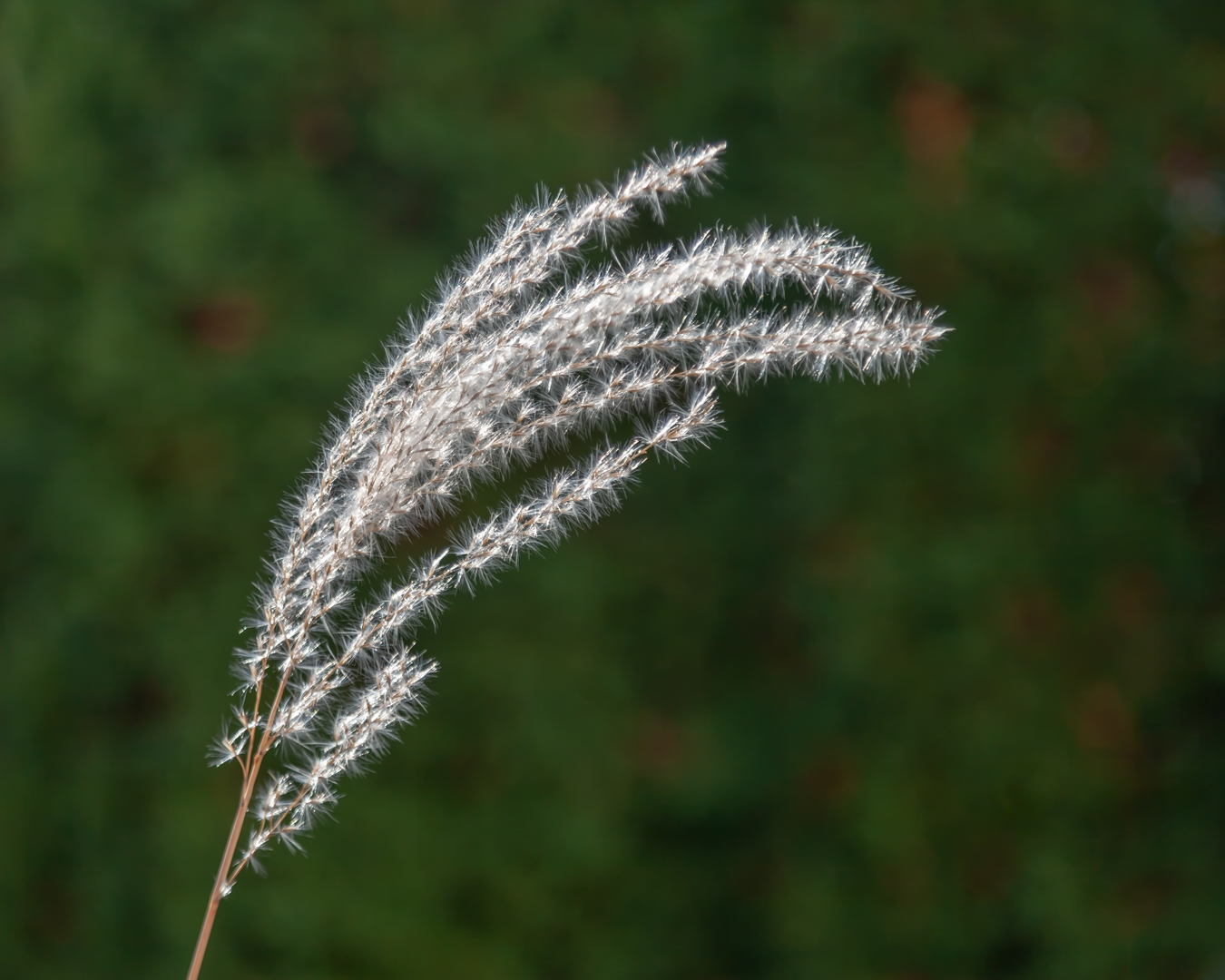The image depicts a single thin, brown branch emerging from the left side and extending upward. This branch, resembling the stem of a wheat plant, is adorned with slender, white, fluffy, wispy strands that look like delicate dandelion seeds, suggesting a fibrous texture. These strands catch the light and appear as though they could be easily blown away by the wind. The branch has several smaller offshoots with tiny leaves that bear a resemblance to soft, fabric-like pipe cleaners. The background, out of focus, hints at a sunlit outdoor scene with dense foliage in varying shades of green and occasional tan splotches, contributing to a vibrant yet blurred natural setting.